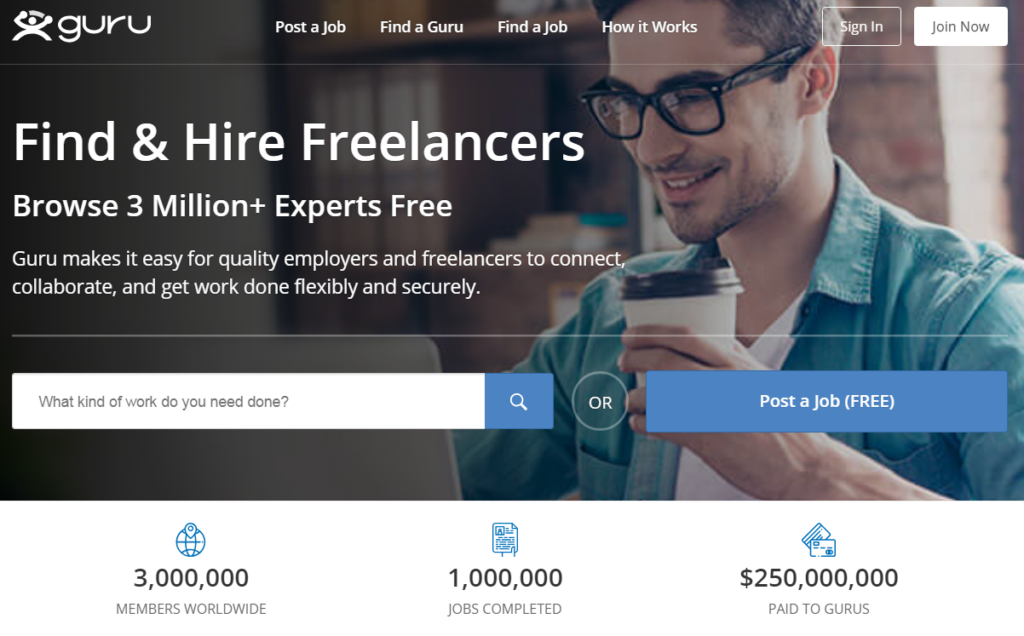The image depicts a detailed and structured layout involving multiple elements. Predominantly, the image features a watch face in a dark black hue, set against the backdrop of an office space. On the right side of the image, a man with short hair and bushy brown eyebrows sips coffee while looking at a gray laptop. He wears black-rimmed glasses and a small mustache, along with a teal dress shirt over a white undershirt. The man holds a white cylindrical coffee cup with a black lid.

On the left side of the image, there's a logo of a man with outstretched arms, accompanied by the text "Guru." At the top are navigation tabs in bold white text labeled: "Post a Job," "Find a Guru," "Find a Job," and "How It Works." To the right of these tabs are two buttons: a semi-transparent "Sign In" button in white text, and a solid white "Join Now" button with black text.

Below these elements, a bold header in white reads "Find and Hire Freelancers," followed by another bold line stating, "Browse 3 Million+ Experts Free." Further down, it says, "Guru makes it easy for quality employees and freelancers to connect, collaborate, and get work done flexibly and securely."

Beneath this description are two rectangles. The first, predominantly white, asks, "What kind of work do you need done?" in black text, accompanied by a blue square with a white magnifying glass encircled in the center. The second rectangle is dark blue with bold white text that reads, "Post a Job," followed by "FREE" in capital letters and parentheses. 

Below these rectangles are various symbols: an image of the Earth with a pin, captioned "3 Million Members Worldwide" in black text; a piece of paper with the letter "A," captioned "1 Million Jobs Completed"; and two overlapping credit cards, captioned "250 Million Paid to Gurus."